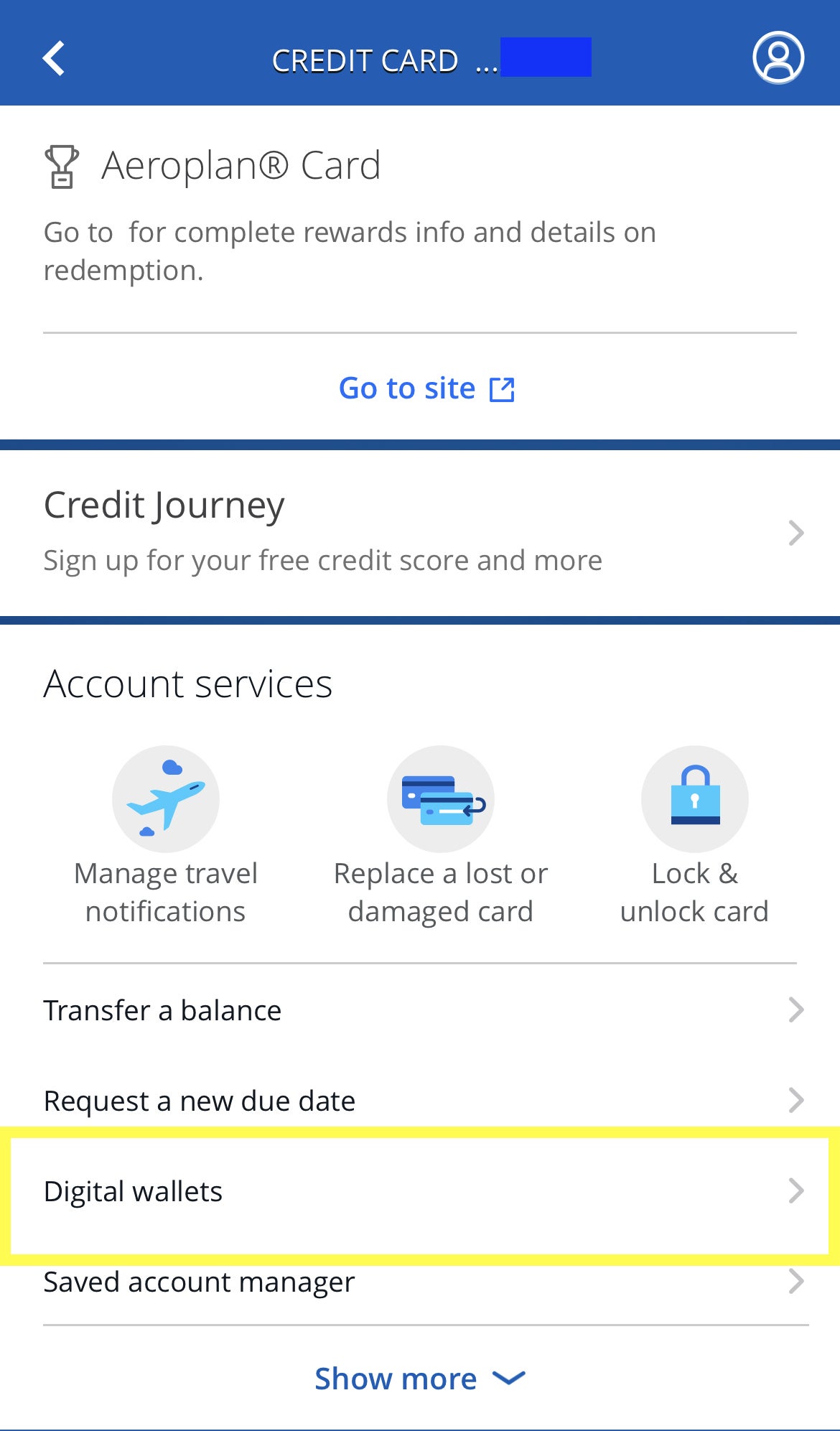The image depicts a familiar user interface commonly seen on financial or credit card management websites. At the top left, there is an arrow icon pointing to a credit card, suggesting an action or navigation related to the card. On the top right, there is an icon representing a user account, depicted as a generic person silhouette.

In the center, the main heading reads "Credit Journey," followed by a subheading labeled "Aeroflam Card." The interface seems to be divided into several segments: "Credit Journey," "Account Services," and a highlighted section called "Digital Wallets."

- **Credit Journey:** Promotes the opportunity to sign up for free credit score access and other services, with a clickable arrow for more information.
  
- **Aeroflam Card:** Provides options for complete rewards and information, or the ability to visit the related website.

- **Account Services:** Features three key functionalities:
  - Manage travel notifications (icon with a plane).
  - Report or replace a lost or damaged card (icon with two cards being switched).
  - Lock and unlock your card (icon with a lock).

Additional options under this section include transferring a balance, requesting a new due date, and managing digital wallets, which is the pre-selected option.

At the bottom of the interface, a "Show More" button is available for users to explore additional features if they haven't found what they are looking for yet. The overall design prioritizes easy navigation and access to various credit card management tools and services.